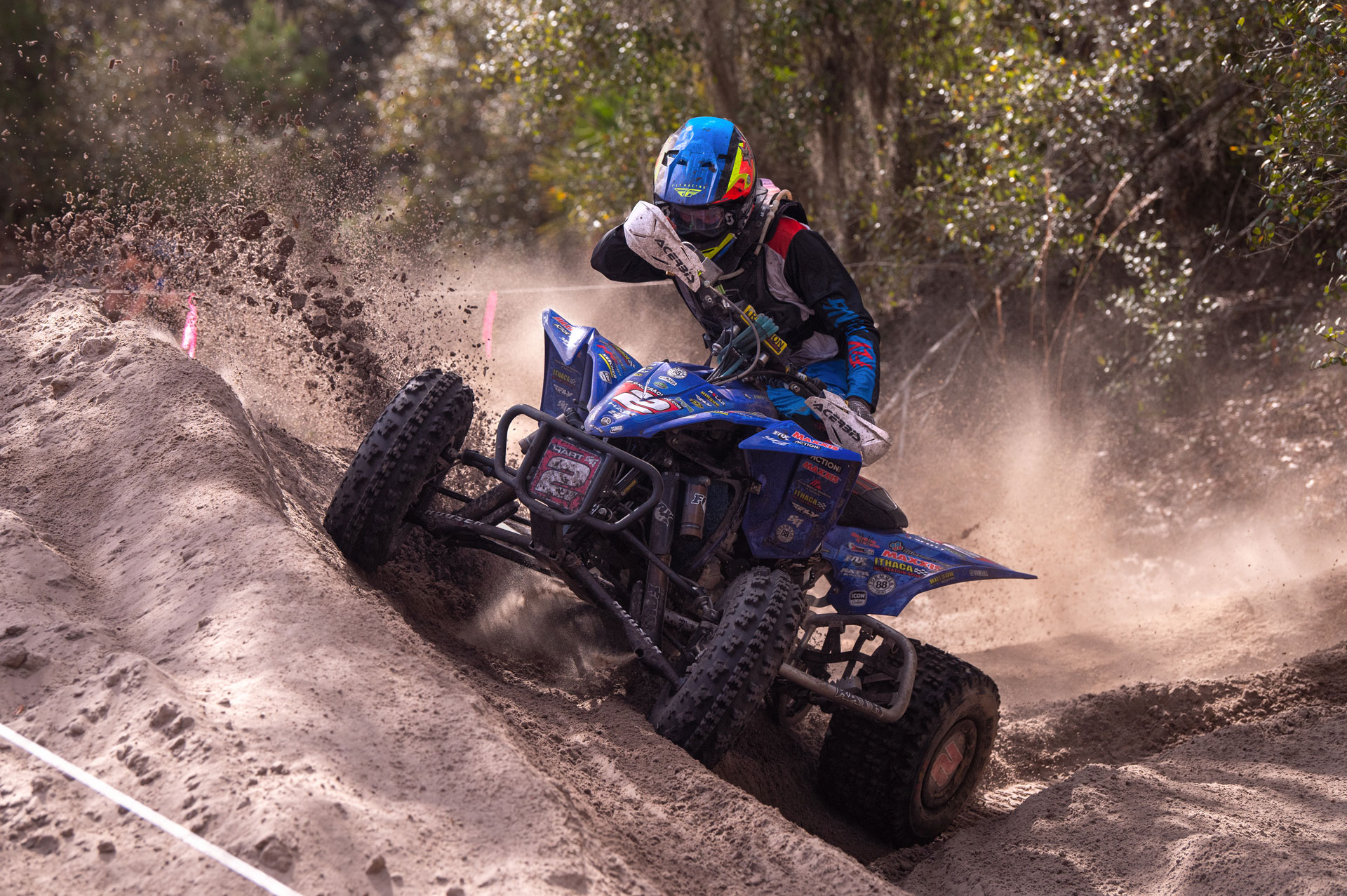This image captures an ATV biker navigating a steep, sandy dirt hill on a challenging, rugged course. Centered in the frame and horizontal in alignment, the rider is depicted in mid-action, appearing precariously close to wiping out as he maneuvers the incline, which is at least a 45-degree angle. The blue ATV with prominent tread on its black wheels shows considerable effort against the incline, kicking up dust and dirt in its wake. The rider is fully geared up, wearing a protective outfit consisting of a black and blue suit accented with neon green, orange, red, and white trim. His blue helmet, adorned with red, yellow, and white details, complements his attire. The setting is unmistakably outdoors, with trees and plants dotting the background, establishing a vibrant yet rugged wooded environment. Dust is seen spiraling behind the ATV and dirt is flung to the upper left, emphasizing the dynamic motion of the scene.